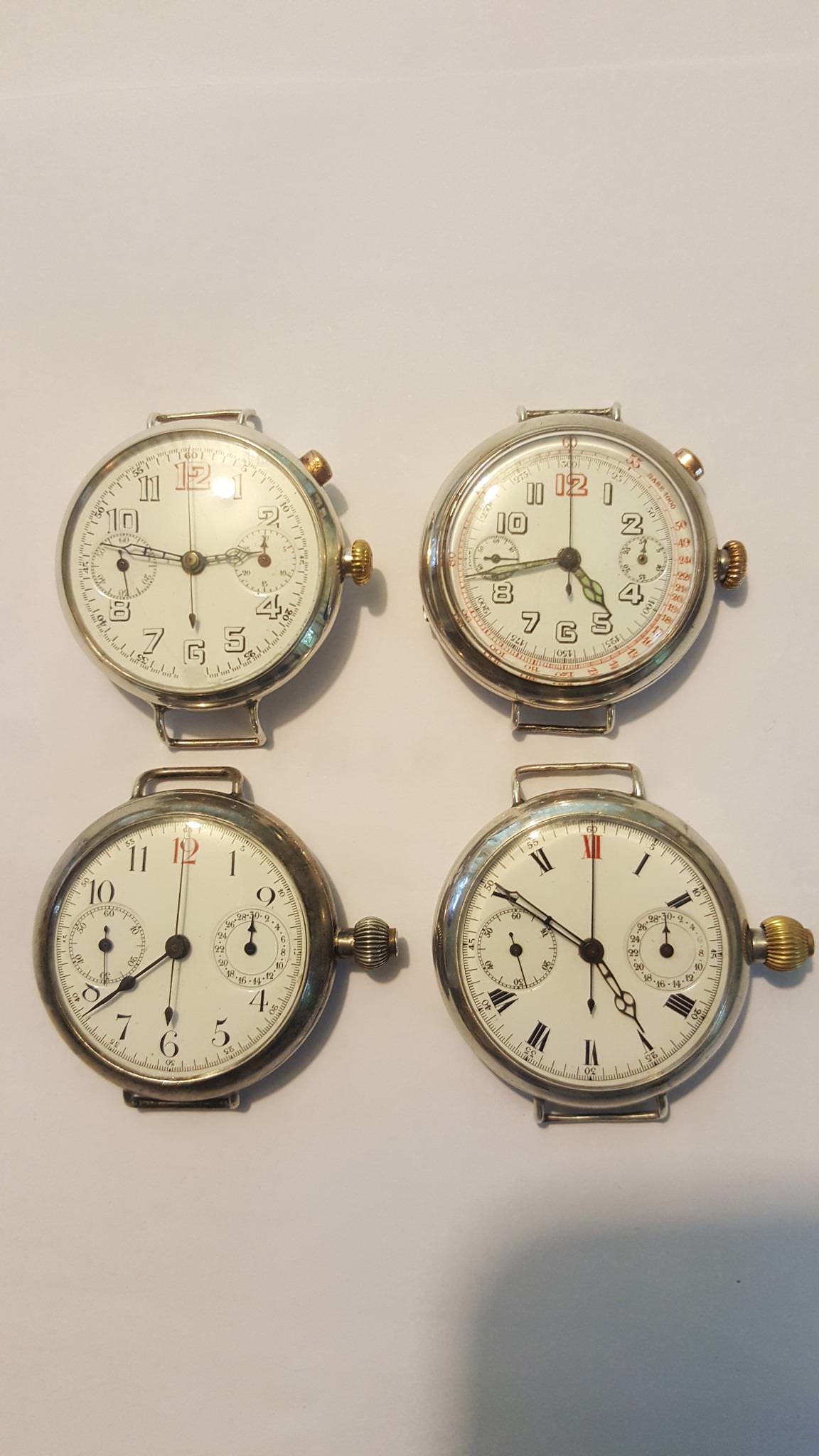This image depicts four vintage wristwatch faces set against a creamy white background, each showcasing elaborate details without their bands. Arranged in two rows of two, the upper left watch features a silver-toned frame and a white background, with the number 12 marked in red. Its silver case includes two buttons on the right side. To its right, the second watch also has a silver-toned frame, a white background with a red-trimmed dial, and a red 12, complementing the similar dual buttons. The bottom row's left watch mirrors the top-left; a silver outline with a white face and a red 12, yet housing a single button on the right. Lastly, the bottom-right watch stands apart with Roman numerals on a white face. Its silver casing has accents of gold on the winding handle, and a single side button. This detailed assembly of watches, harmonized by their metallic silver outlines and shared vintage aesthetic, is accented by the unique touch of red marking the 12th hour on each face.